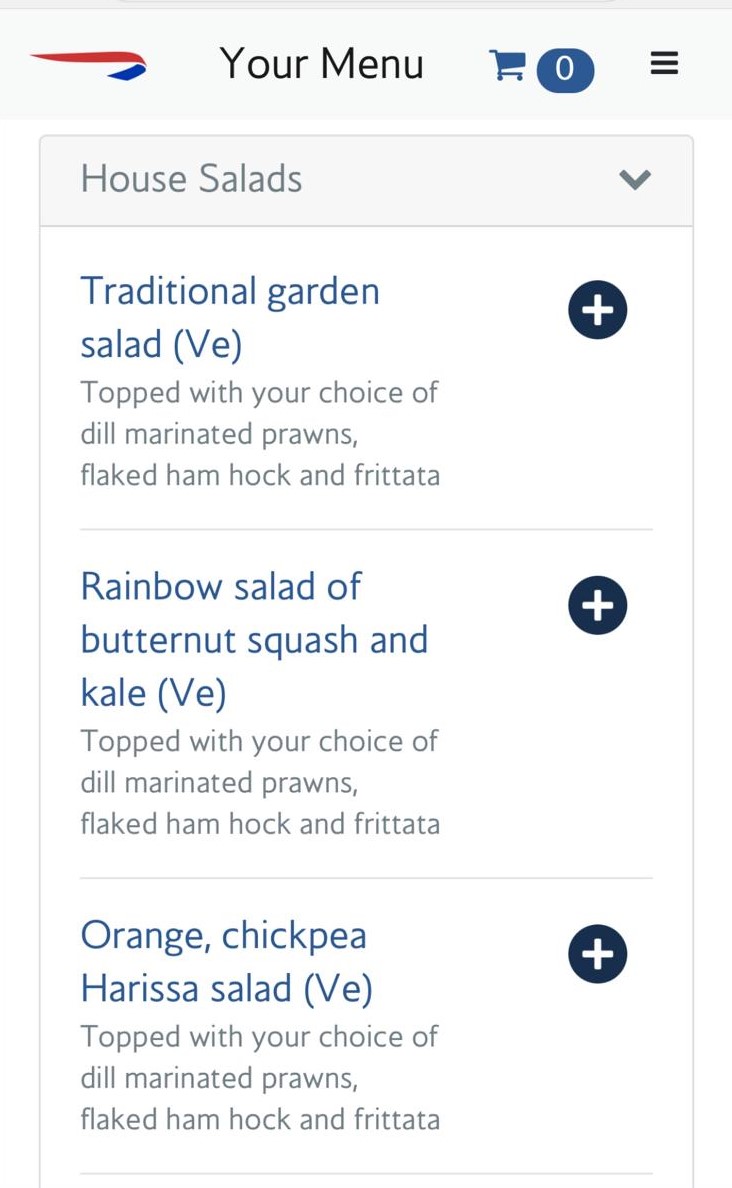The image appears to be a digital food menu interface. At the top of the menu, there is a header that reads "Your Menu" accompanied by a shopping cart icon with a "0" indicating no items have been added yet. 

On the upper left corner, there is a distinctive logo: a ribbon-like design with a larger red section and a smaller blue section.

On the upper right corner, there's a black hamburger menu icon, which typically indicates a clickable menu for additional options or navigation. Directly below this icon, the text "House Salads" is displayed.

The menu lists several salads under this section:
1. Traditional Garden Salad (VE)
2. Rainbow Salad of Butternut Squash and Kale (VE)
3. Orange Chickpea Harissa Salad (VE)

Each salad has a gray subtext suggesting additional toppings: "Top with your choice of dill-marinated prawns, flag time hock, and frittata." This text seems to apply to all the listed salads, despite the toppings being incongruous with some of the salad names.

To the right of each salad option, there are circular buttons featuring a white plus sign, presumably for adding the selected item to the cart.